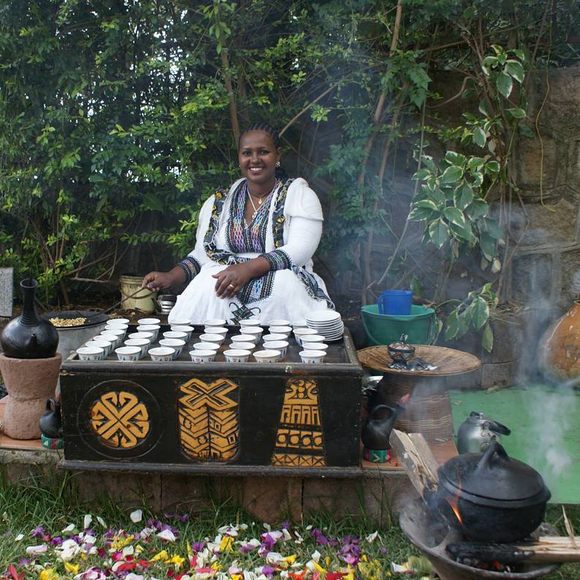In this vibrant outdoor scene, a smiling Black woman sits at the center, preparing a meal. She is dressed in a traditional white dress adorned with a striking blue pattern around the sleeves and neckline. A distinctive blue shawl with colorful tassels drapes around her shoulders and midsection, adding a touch of vivid color to her attire. Her left hand rests gracefully on her lap, showcasing a gold wedding band, while her right hand holds a ladle, stirring a pot of stew. 

In front of her, there is a black wooden box with elaborate gold etchings and a selection of small white teacups neatly lined on top, alongside stacked saucers. To her right, a green bucket containing a blue pitcher is positioned near a flat wooden structure holding another pot. Further right, a piece of metal with two wooden sticks protrudes upwards, their tips aflame, supporting a black pot over the fire.

Behind her, lush greenery composed of tall trees and vines envelops the scene, with patches of blue sky visible through the leaves. Colorful flowers, including hues of purple, white, red, and yellow, sprout from the grass at her feet, enhancing the natural beauty of the setting. Smoke wafts gently from the cooking area, mingling with the bright daylight that illuminates the picturesque tableau.